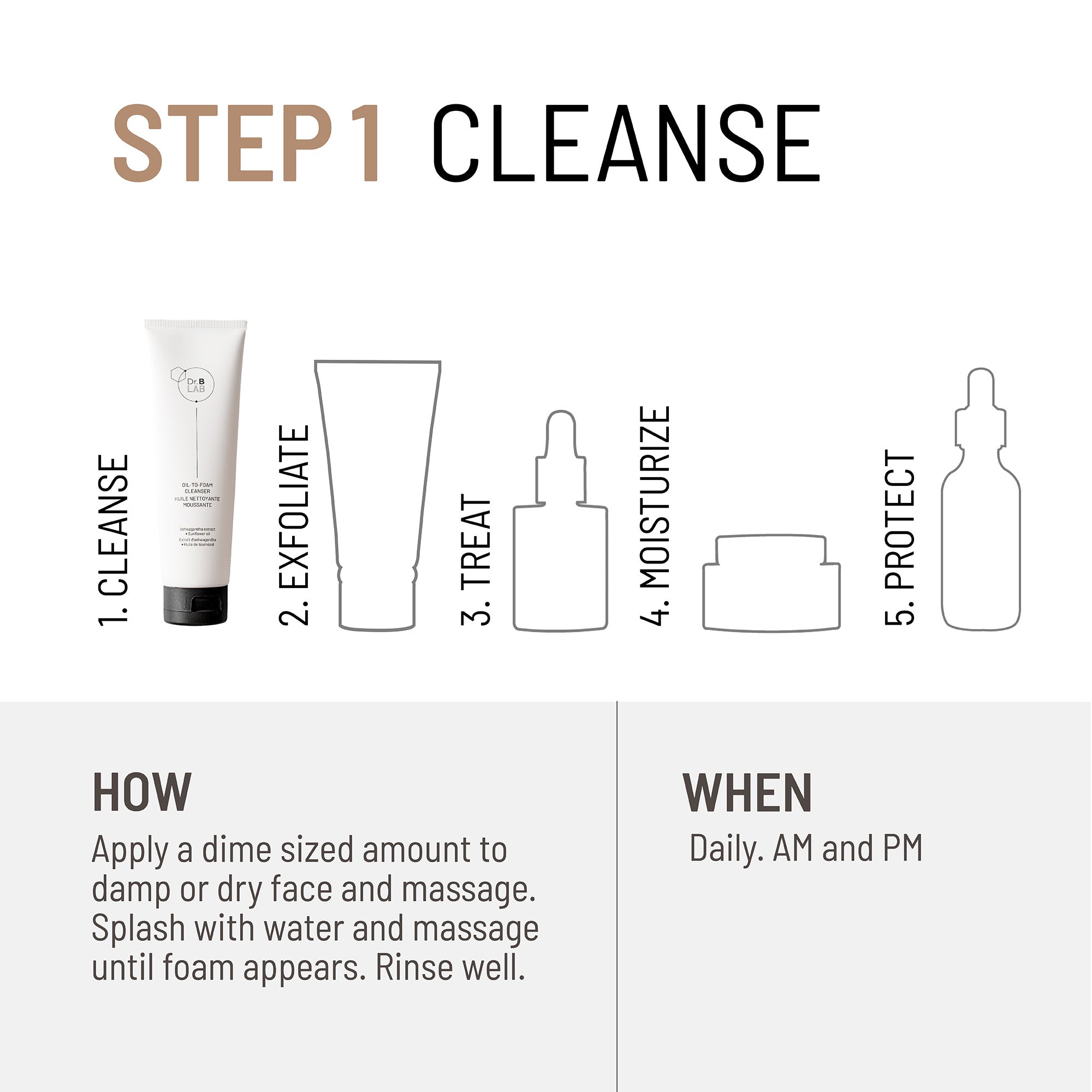This detailed black and white illustration outlines a comprehensive five-step facial care routine. At the top, "Step 1" is written in tan letters, with "Cleanse" in equally large black letters to the right. Below, each step is depicted with corresponding products:
1. **Cleanse** – A white tube with a black cap, likely a facial cleanser.
2. **Exfoliate** – Illustrated by an outlined tube.
3. **Treat** – Represented by a small jar with a dropper top.
4. **Moisturize** – Indicated by an outlined jar.
5. **Protect** – Marked by another small jar outline.

At the bottom, detailed usage instructions explain the cleansing process:
- _How_: Apply a dime-sized amount to damp or dry face, massage, splash with water, and continue massaging until foam appears, then rinse well.
- _When_: Daily, both in the a.m. and p.m.

This guide is designed for anyone looking to maintain and protect their facial skin through a sequential treatment regime.